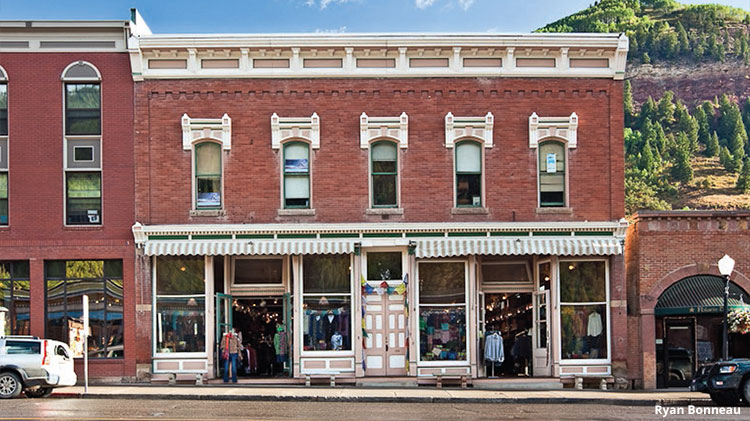This detailed color photograph captures an old-fashioned red brick building set against a mountainous background with trees. The primary building is two stories high, featuring five windows across the second floor and a white ornate roof lining. The ground floor hosts two shops, each with its own awning, displaying mannequins and clothing racks outside their respective open doors and windows. The building has a duplex-style layout with a door in the middle flanked by a window, door, and window sequence on either side. 

Located to the left of this main building, there is an old-fashioned lamppost. To the right, the photo includes a shorter, one-story red brick building with a green awning and a street lamp in front of it. Part of a black car is visible parked at the curb in front of the smaller building. Another vehicle is also parked further along the curb. There is signage on the sidewalk, albeit not readable. In the background, the hillsides are dotted with numerous trees, adding to the picturesque setting. At the bottom right of the photograph, the photographer's name, Ryan Bonneau, is credited. 

Overall, this vivid snapshot encapsulates the charm of historic architecture juxtaposed with the natural beauty of the surrounding mountainous landscape.